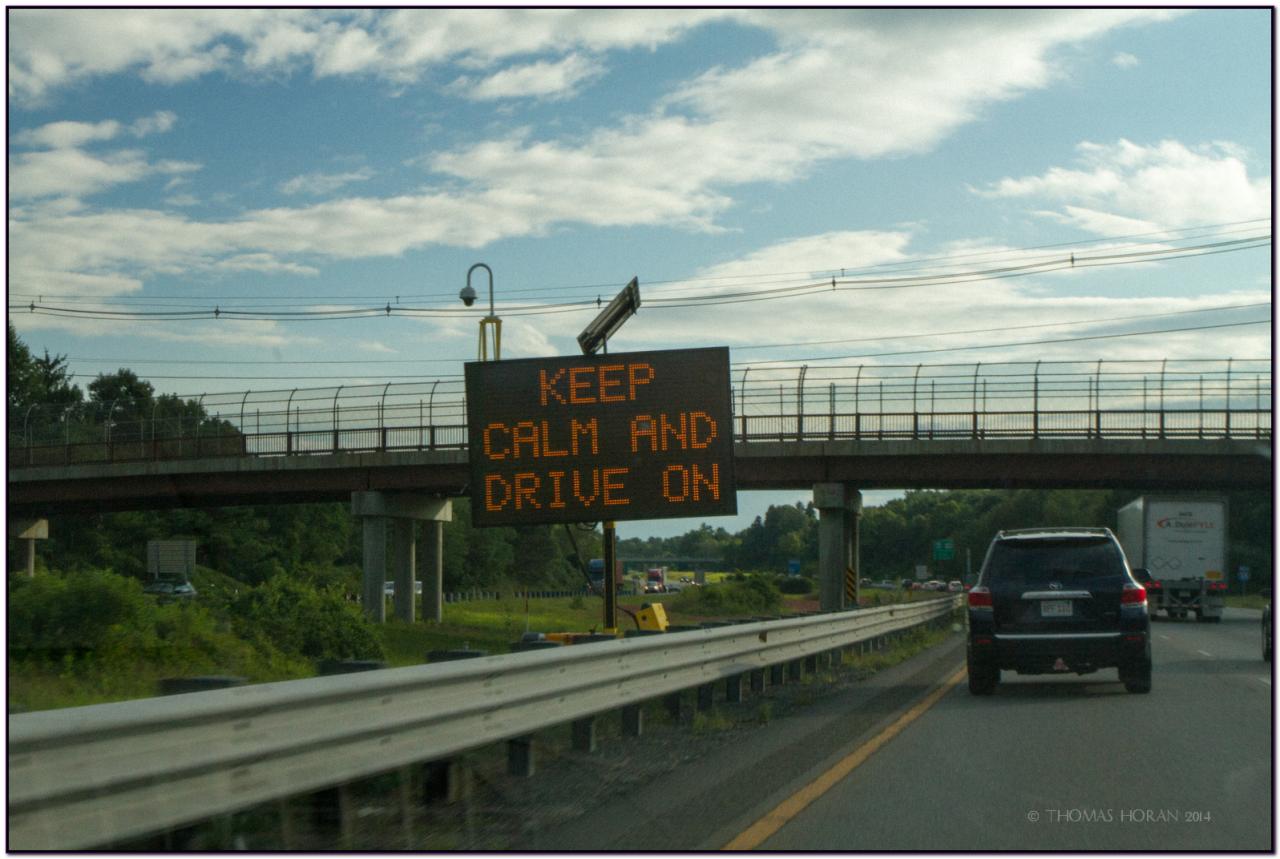The photograph captures a divided multi-lane highway scene with a prominent digital highway sign at the center, emblazoned with "Keep Calm and Drive On" in vivid orange lettering. The sign, rectangular with a slight square aspect, is topped with a solar panel and is supported by a single central post. To the left, there's a light gray guardrail and a yellow line with a rumble strip, beyond which lies oncoming traffic in a wide median. A dark blue Toyota SUV travels in the left lane, while a white tractor trailer marked with red and black logos, including red swish marks and two diamonds, advances in the right lane. Both vehicles are approaching an overhead elevated roadway that crosses the highway, with accompanying power lines visible above. The sky is blue, adorned with feathery clouds, suggesting a clear afternoon. Additionally, visible in the lower right corner is a faint white copyright text reading "Thomas Horan 2014."